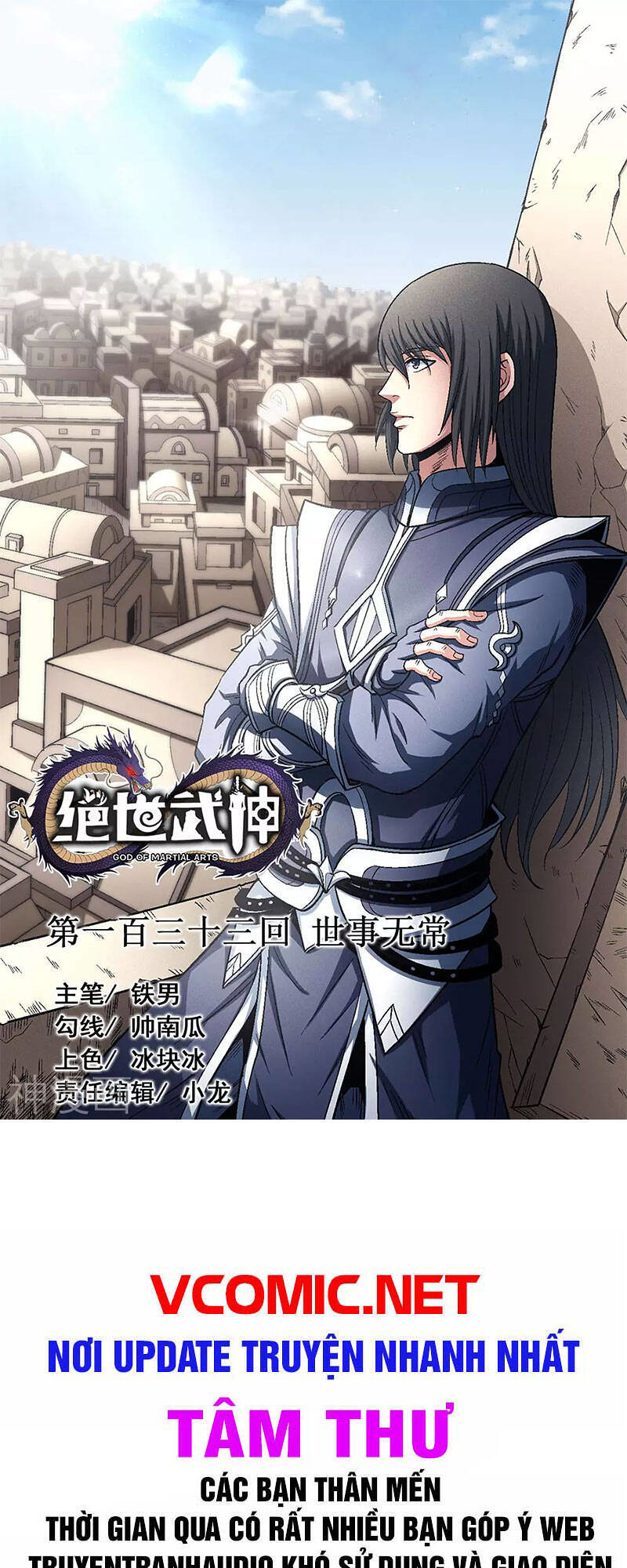This poster advertises an anime or manga website, prominently featuring an intricately detailed drawing of a character with long, shaggy black hair. The character is dressed in a striking blue and purple outfit with black belts and white trim, exuding an elegant and mysterious vibe. He is leaned against a wall, gazing over a cityscape composed of numerous buildings in shades of tan and white. The sky above is a vivid blue, adorned with white clouds and the sun positioned in the top left corner. At the bottom left of the image, a cluster of Chinese characters is inscribed. Beneath this, the URL "vcomic.net" is displayed in bold, red text, followed by blue and pink text lines underneath, and a final line of small black text in a different Asian language, possibly Vietnamese. This poster conveys a vibrant and dynamic atmosphere, hinting at a rich, narrative-driven experience offered by the website.